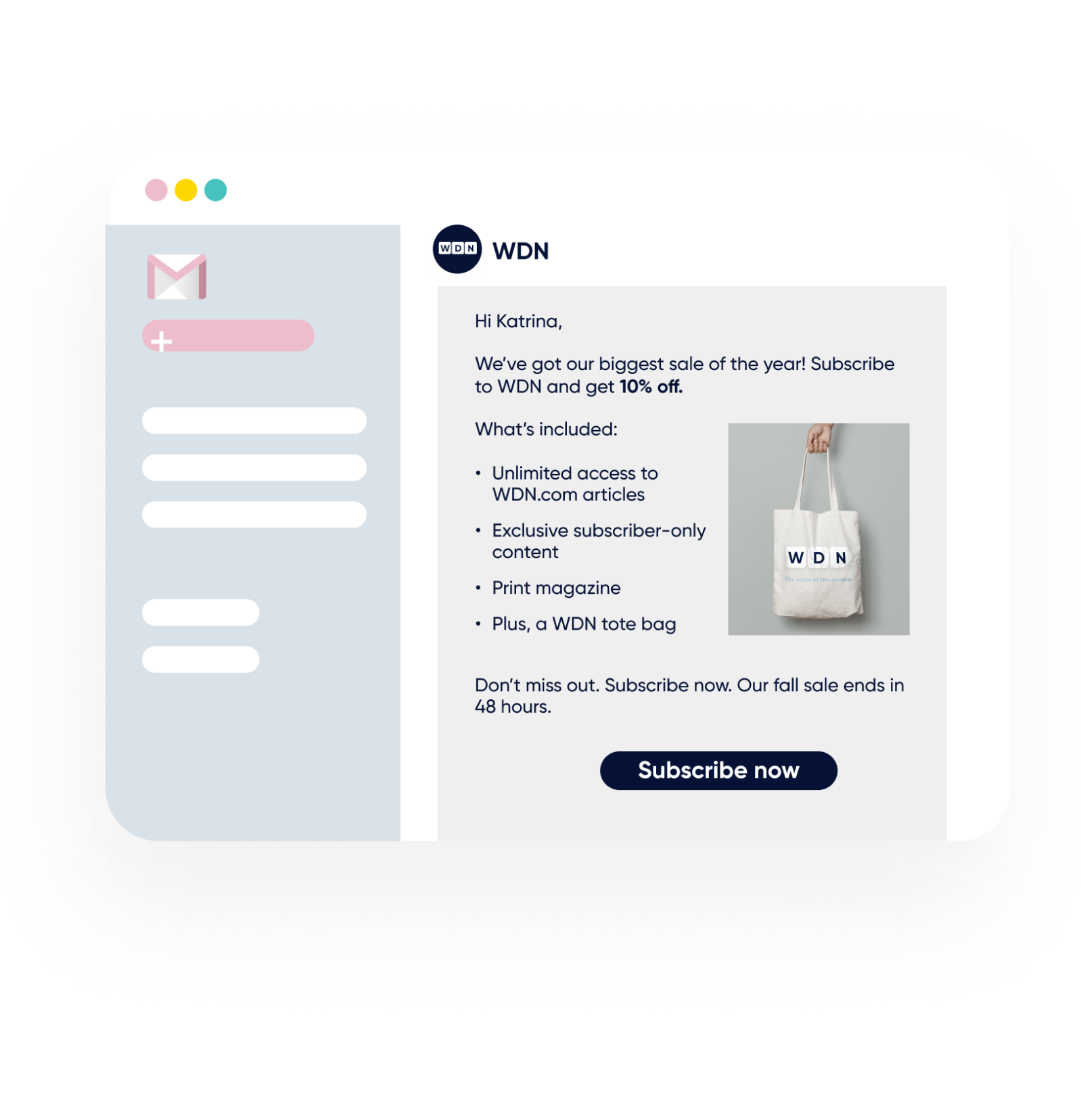Here's a detailed and cleaned-up caption for the image:

This screenshot, likely taken from a tablet, features two main sections. On the left, there's a box displaying a Gmail icon - an envelope outlined in pink. Above this box, three small circles are visible in light purple, yellow, and teal.

The box on the right presents an email promotion from WDN. The email greets the recipient with "Hi Katrina," and announces their biggest sale of the year. It invites the recipient to subscribe to WDN to receive a 10% discount. The content details the promotion, although some parts are summarized as "blah blah blah." Below the promotional text is a prominent "Subscribe Now" button.

The email also includes a single photo: an arm holding a white tote bag marked with the letters "WDN." There is additional light wording across the bottom of the tote bag, but it is not clearly visible. This tote bag image is the only photograph featured in the screenshot.